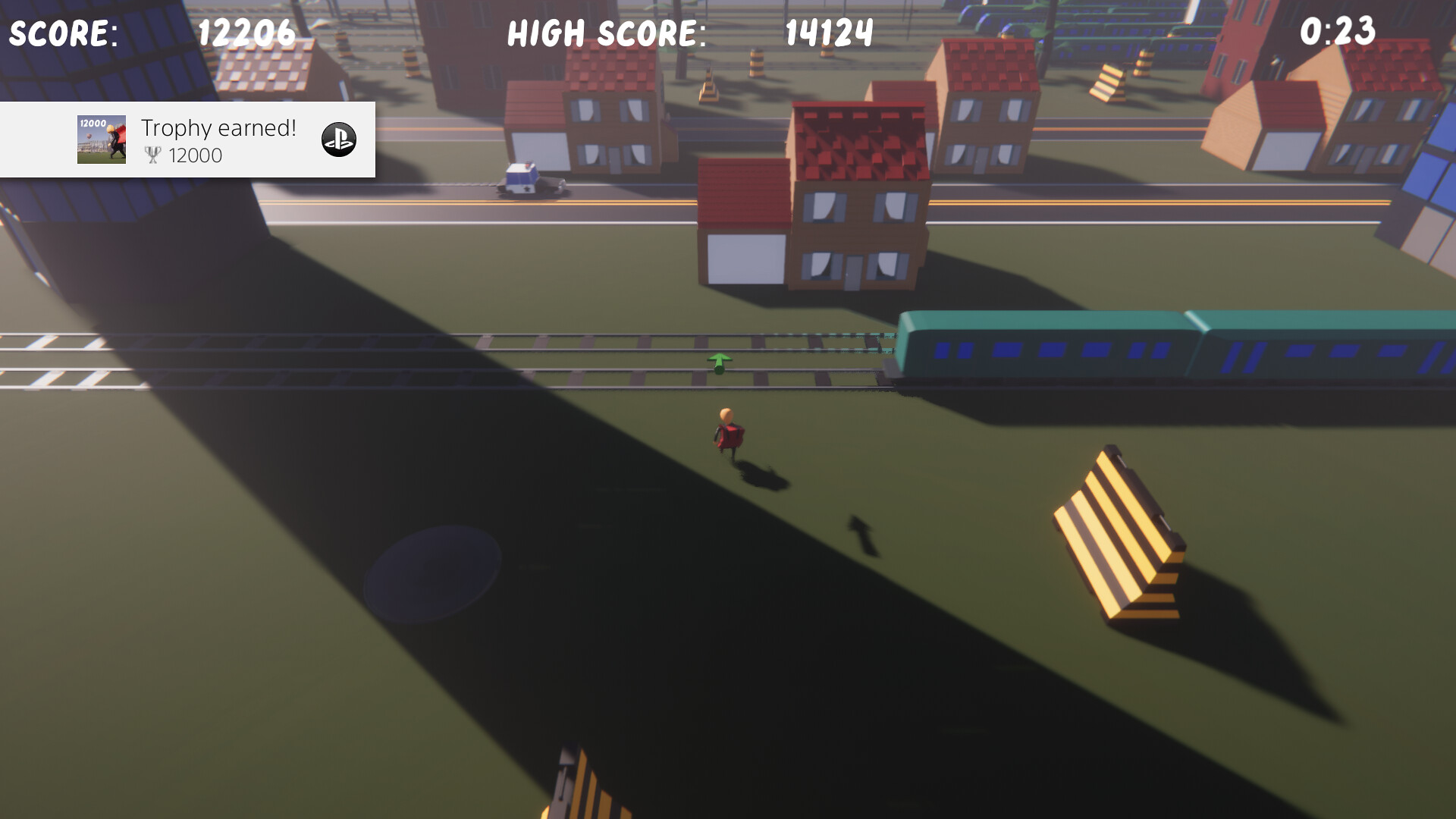This image is a screenshot from a video game set in a quaint little town. The scene is vividly detailed with lush green ground, houses lining the streets, and a railroad track running horizontally across the screen. In the center, a small character equipped with a large red backpack appears to be preparing to cross the railroad tracks. Further ahead, houses continue to dot the landscape, leading up to a street where a miniature police car is driving from left to right. At the top of the screen, the player's score is prominently displayed as 12,206, with the high score noted as 14,124. The in-game timer shows that the player has 23 seconds left, and a trophy icon indicates that they have already earned an achievement. The interface confirms that this game is being played on a PlayStation console.